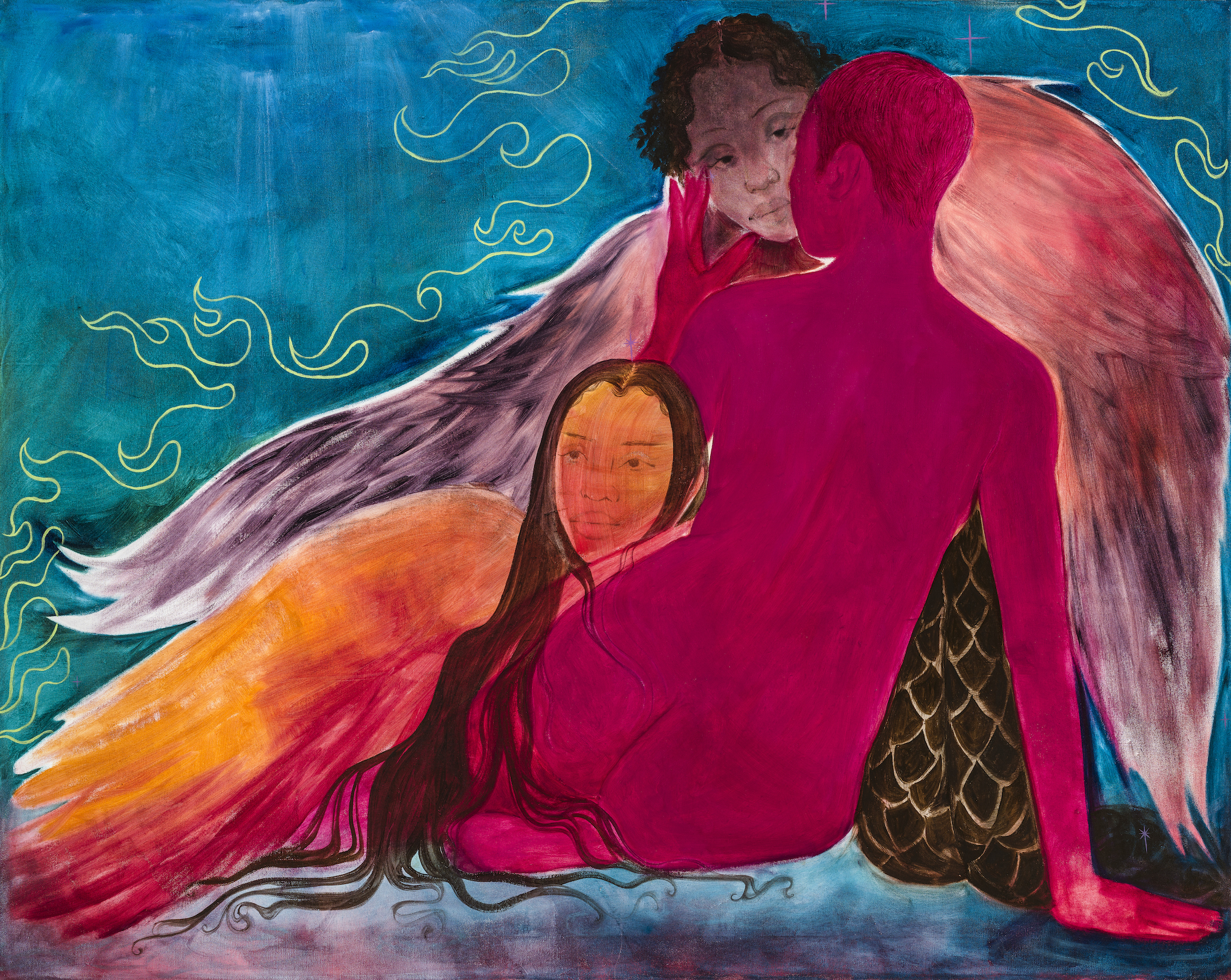This striking and vibrant painting features three figures set against a mesmerizing blue background interspersed with yellow, flame-like outlines. In the center is an African-American man with curly black hair extending to his ears. He dons black attire paired with white checkered, diamond-patterned pants, and boasts angelic wings that blend hues of pink, black, and white. He is seated, his legs appearing somewhat scaly, and he engages directly with the viewer. A second figure, possibly another woman, leans against this central figure on his left side, her long brown hair cascading and adorned with yellow and orange feathers, giving the impression of wings. She clutches his head tenderly. On the far right is a nude woman with a striking pink complexion, supporting herself with her right arm. Her left hand rises to her face, meeting the face of the central figure, creating an intimate interaction. Her figure is integrated into the composition with her body language leaning towards the right. This intricate and colorful tableau, surrounded by a visually arresting backdrop of swirling blue and yellow flame-like elements, creates a sense of an ethereal and underwater-like realm, enhancing the painting's beauty and depth.